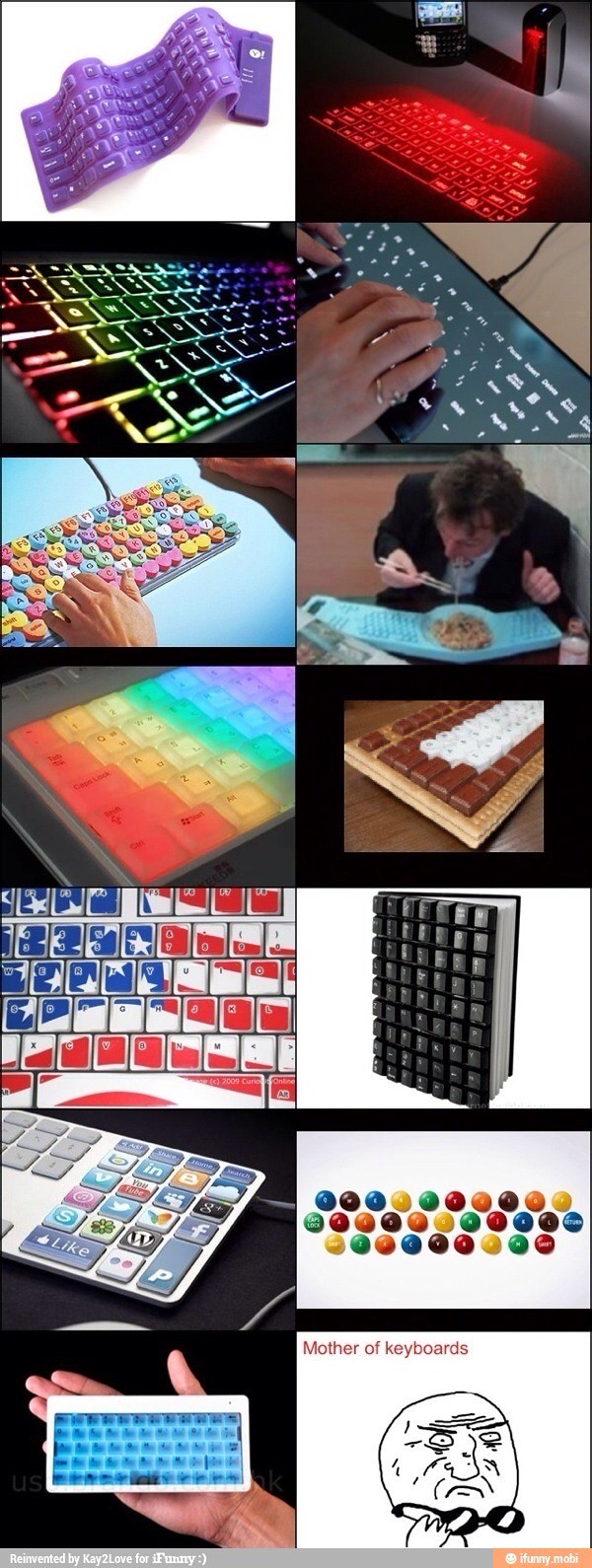The image is a vertical collage composed of 14 diverse images of creative and unique keyboards, arranged in two columns with seven rows each. Starting from the top, the first image features a purple silicone keyboard that appears crinkled, more as an art piece than a functional device. This is followed by a vibrant red digital keyboard and a rainbow-colored keyboard with illuminated backlighting. Next is an ultra-flat, touch screen-like keyboard, and a whimsical candy heart keyboard. Continuing down, there's a teal keyboard with a bowl in the center, from which a man is eating. Another image showcases a second rainbow backlit keyboard. Next is a s'more-themed keyboard with chocolate-like casing and white keys. There’s also a patriotic keyboard adorned with the American flag, followed by an image of buttons glued to a book cover, and a keyboard displaying a series of icons. An M&M-themed keyboard follows, then a miniature keyboard that fits in the palm of your hand. Lastly, the final image at the bottom right is a meme from the Rageface era, depicting a wrinkled, frowning face with glasses in hand, captioned "Mother of Keyboards," indicating the collection's variety. The collage not only displays an array of unique designs but also highlights the creativity and humor in keyboard customization.